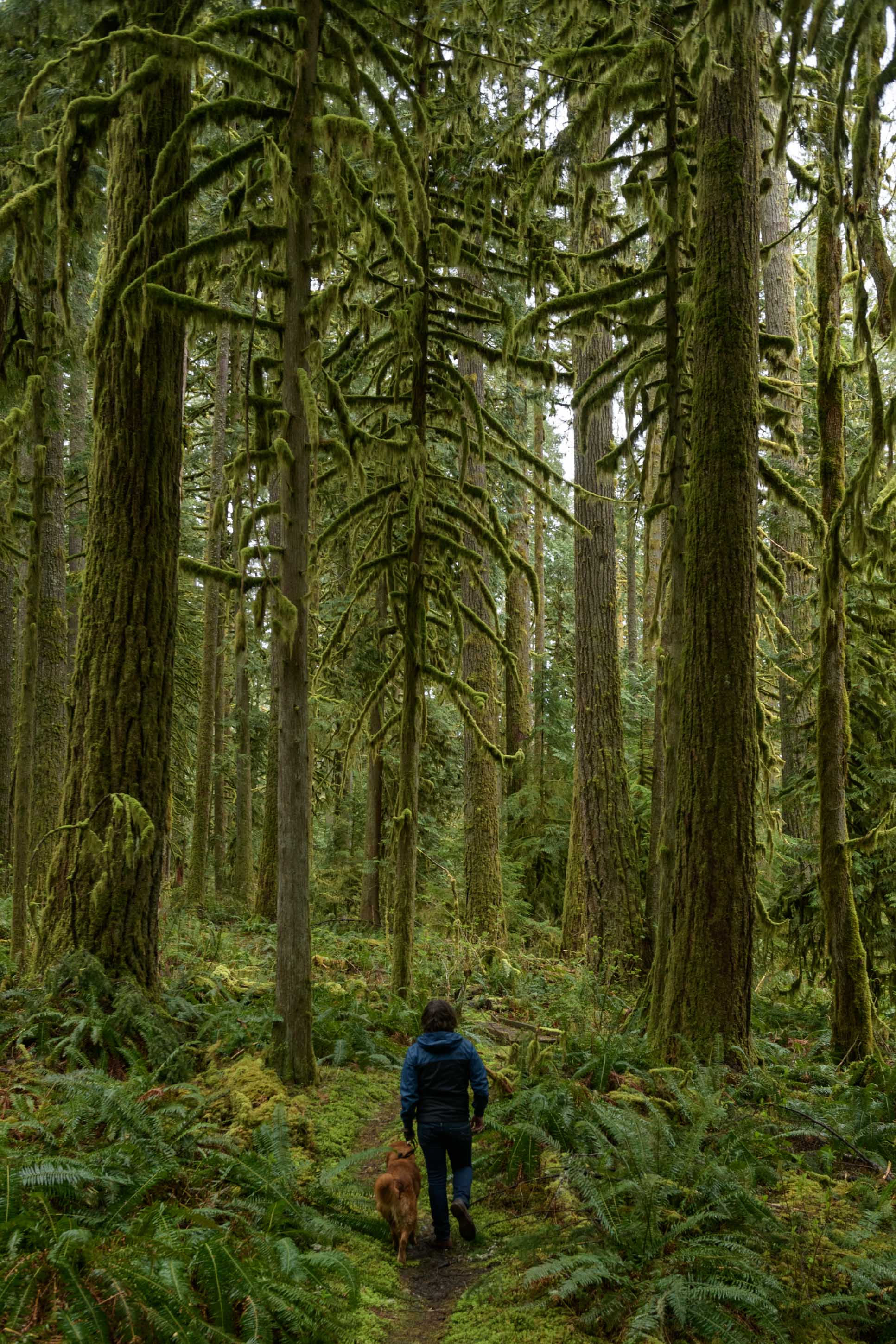In this image, a man, dressed in a blue tracksuit with a hoodie and jeans, is trekking with his golden retriever along a narrow dirt trail in a dense, forested area. He has shoulder-length black hair and is walking away from the center of the photograph towards the deeper parts of the forest, holding his dog on a leash. The forest is characterized by its very tall and thin tree trunks, possibly well over 100 feet tall, which are heavily covered in moss and small green plants. The trees have fir-like, pine-style branches that contribute to the thick vegetation both on the trees and the ground below. The forest floor is abundant with lush, bushy plants and brush, indicating a rich and dense undergrowth. This scene, likely set in the North Pacific Northwest or a similar North American or European forest, exudes a serene atmosphere in the daytime, indicated by the sunlight filtering through the tree canopy, casting shadows and illuminating the trail. The area appears mountainous and ancient, with a sense of isolation as the man and his dog are the only beings visible in the frame, highlighting the tranquility and seclusion of their nature walk.